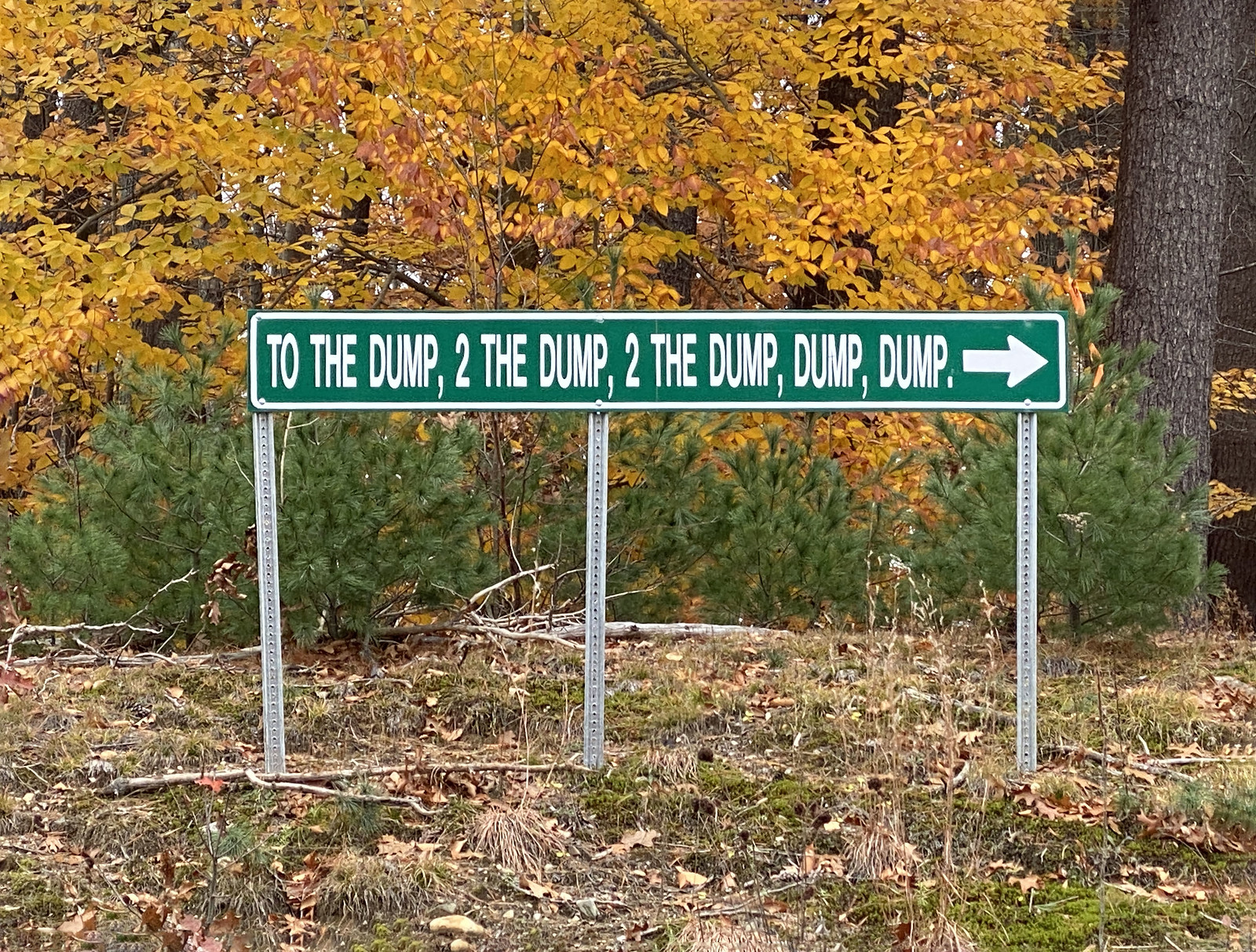The image showcases a prominent street sign situated on the side of a road, supported by three metal poles. The sign, which dominates the center of the image, features a green background with a white border. The white text on the sign reads: "To the dump, to the dump, to the dump, dump, dump." A white arrow points to the right, indicating the direction.

The ground below reflects the autumn season, with patches of brown from dying plants interspersed with green grass. Short green trees or bushes are visible in the foreground, while trees with yellow leaves are seen in the background. To the right, several brown tree trunks add to the fall atmosphere of the scene.